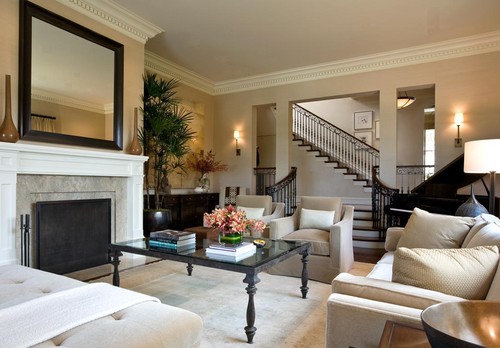This cozy and elegantly designed living room features a sunken layout accessible via five steps adorned with curved black wrought iron handrails. Prominently positioned to the right as you descend is a grand black piano. The focal point of this space is a sophisticated fireplace situated in the bottom left corner, boasting a white mantle above which hangs a large mirror encased in a sleek black frame. Surrounding the fireplace is chic gray marble, complemented by black fireplace tools hanging to its left.

Central to the room is a large coffee table with a black metal frame and a glass top, adorned with three neatly arranged books and a vibrant bouquet of orange flowers in a green glass vase. The seating area includes a tan couch that harmonizes with lighter beige walls, further accentuated by matching throw pillows.

The high ceilings are smooth, embellished with intricate carvings along the border. Notably, an upstairs staircase with dark brown wooden steps and a matching guardrail adds to the grandiose feel of the room. The staircase wall is a crisp white, contrasting with an adjacent dark wood desk. The space also features additional seating, lamps, and a few strategically placed green plants which introduce a touch of nature. The overall color scheme of beige, brown, and black, combined with ample natural light and the warmth of the furnishings, creates a modern yet inviting atmosphere.